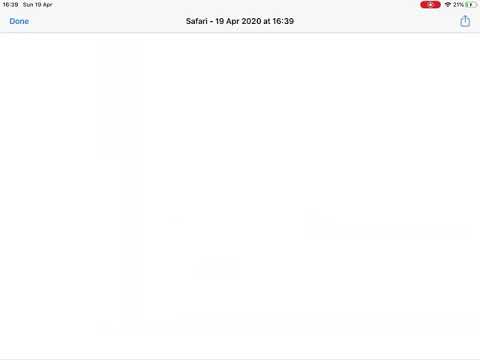The image features a primarily white background with a gray bar stretching horizontally across the top. The bar displays various bits of information: on the left side, in very light gray text, it reads "16:38 SUN 10 April APR." Below that, there are blue or green text elements stating "Done."

Centrally aligned within the bar, it says "SAFARI - 19 APR 2020 at 16:39."

On the right side of the bar, there is a red button featuring a circular symbol, along with text indicating "21%," presumably referring to the battery charge. This portion is noticeably pixelated and difficult to read. The rest of the screen below the bar is entirely blank and white, with the information on the gray bar being the only content visible. 

The image quality is poor, with very low resolution, making it hard to discern certain details. There is an absence of any other contextual clues to determine whether the image is from a phone, computer, or tablet, beyond the mention of Safari.